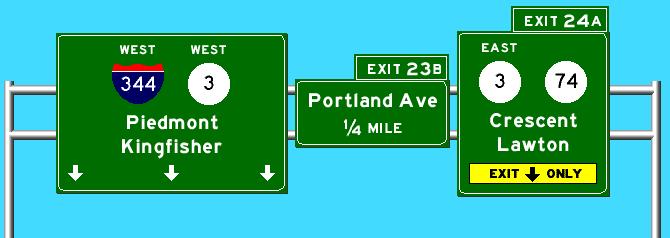This intricate pixelated drawing features a trio of dark green highway signs, evoking a nostalgic feel reminiscent of classic video games like those from Atari. The image likely depicts a screenshot from such a game, capturing the characteristic blocky aesthetic.

On the left, the largest sign reads "West 344" inside a blue and red shield-shaped icon with white lettering. Beneath that, within a white circle, "West 3" is displayed in black text. Below, a directional guide states "Piedmont to Kingfisher" accompanied by three downward-pointing arrows.

The central sign, the smallest of the three, features two rectangular sections. The top section, in a smaller rectangle, says "Exit 23B." Below it, the larger rectangle provides the distance marker "Portland Avenue 1/4 mile," all written in white.

On the right, the medium-sized sign is divided similarly. The upper smaller rectangle reads "Exit 24A." Below, the main portion of the sign indicates "East 374," with the numbers "3" and "74" inside white circles with black text. Underneath, "Creston Lawton" is inscribed in white. The lowest section of this sign is a thin yellow rectangle stating "Exit Only" in black text, accompanied by a downward-pointing black arrow.

This detailed artwork encapsulates the essence of retro gaming through its vintage highway sign imagery.